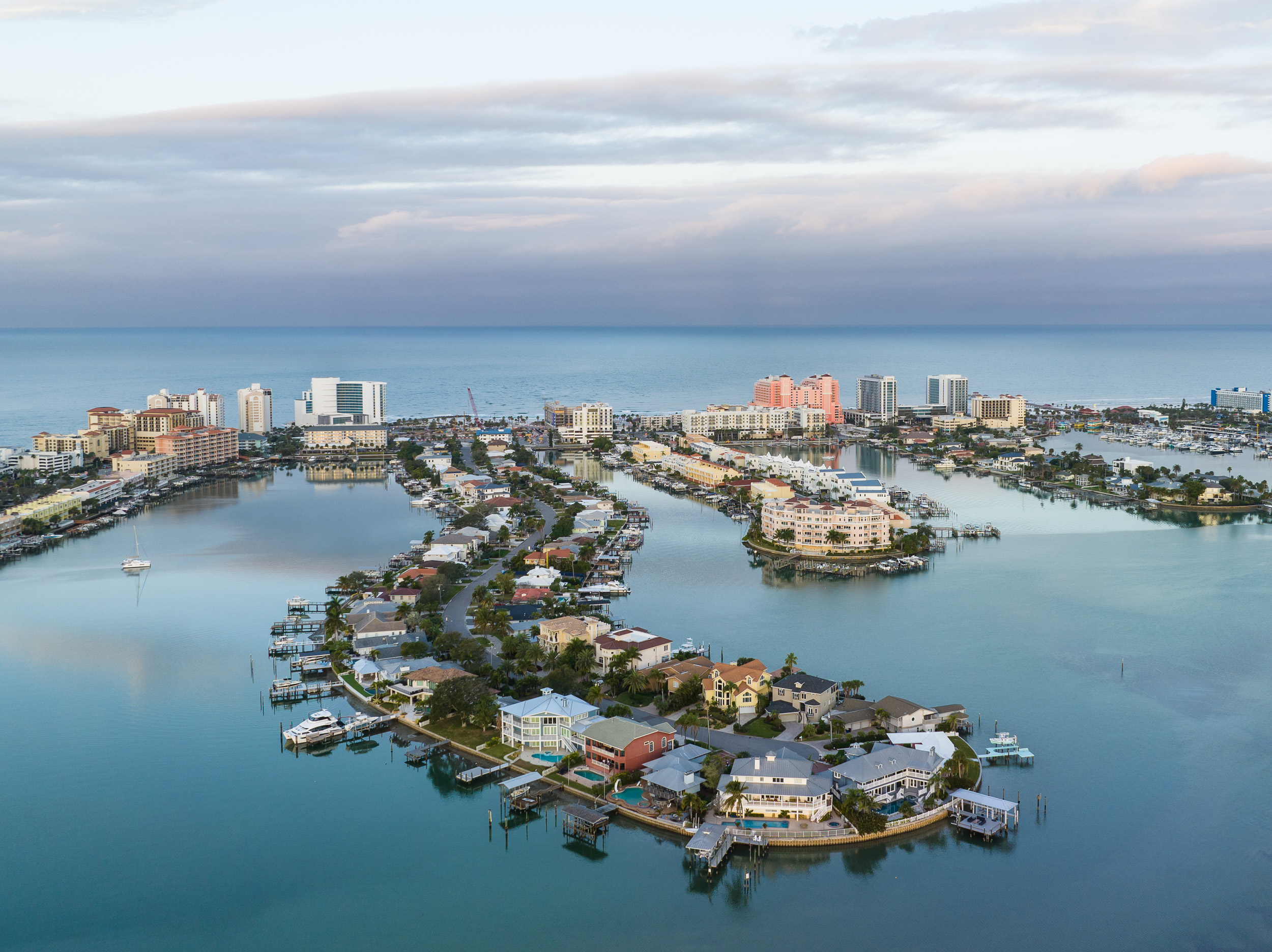A sprawling aerial photograph captures a landscaped sea vista dominated by an intricate network of man-made peninsulas stretching from the middle of the right to the middle left side of the image. These peninsulas cradle large, mansion-style homes, each accompanied by small docks or piers. This elaborate layout appears to branch off a central island, creating an island-like structure teeming with sprawling houses and possibly condominium buildings up to around 10 stories tall. The foreground water is incredibly smooth and calm, with a rich blue shade that extends to the horizon, beyond which lies more of the ocean. The sky above is overcast with hues of pinks and grays, offering a serene backdrop that is slightly hazy but still illuminated by enough sunlight. Several boats drift leisurely on the water, enhancing the tranquil ambiance of the scene. The photograph highlights the harmonious blend of luxurious human habitation against the serene stillness of the expansive ocean.